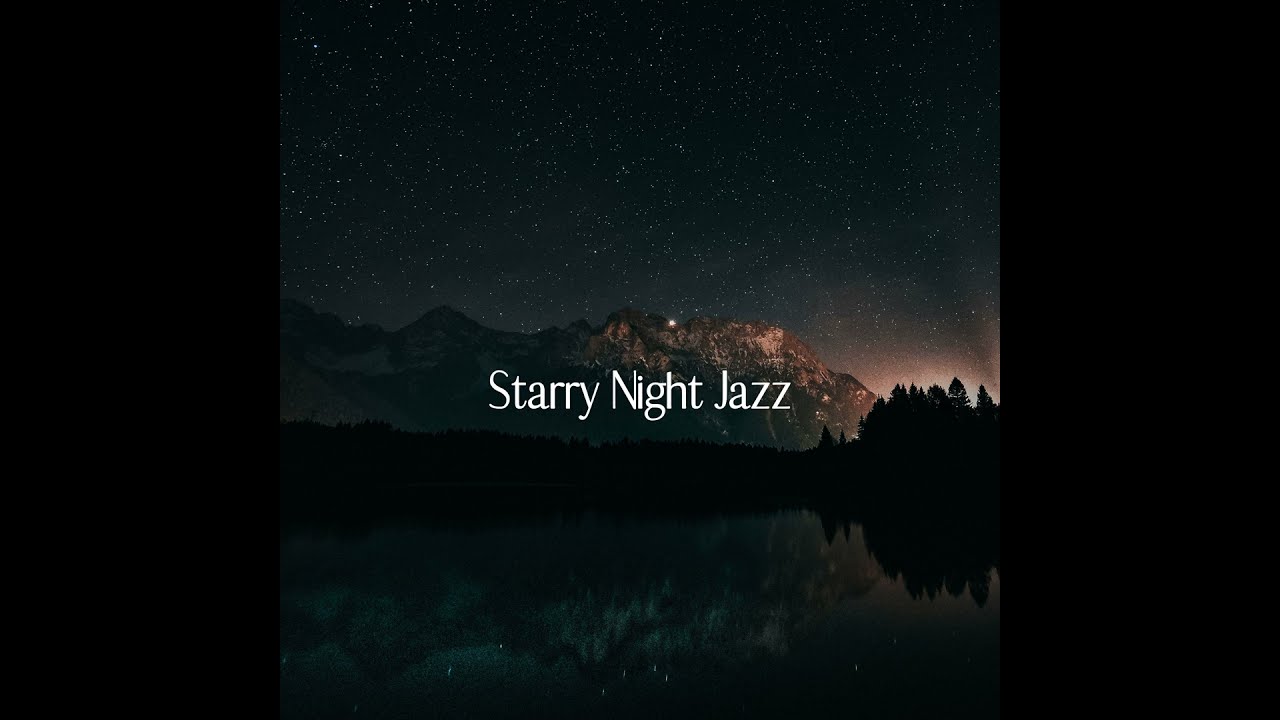This rectangular image, roughly six inches wide by three inches high, mimics the style of a jazz album cover and is primarily focused on nature. It features thick black borders on the left and right sides, adorned with small white sparkles, reminiscent of a starry night. At the center of the image, white text reads "Starry Night Jazz." The top half of the picture showcases a deep blue, star-filled night sky. Beneath the sky lies a dramatic mountain range with dark gray rocks, some peaks capped with white snow. There is a line of silhouetted trees below the mountains, with notably taller trees on the right side. A glowing light beneath these trees creates an illuminated effect on the right side of the mountains, suggesting a setting sun. At the bottom of the image, a crystal-clear lake perfectly reflects the entire scene above, including the stars, mountains, and trees. The color palette includes deep blue, black, gray, white, tan, brown, and hints of green, all contributing to a serene, nocturnal landscape that reflects the album's theme.